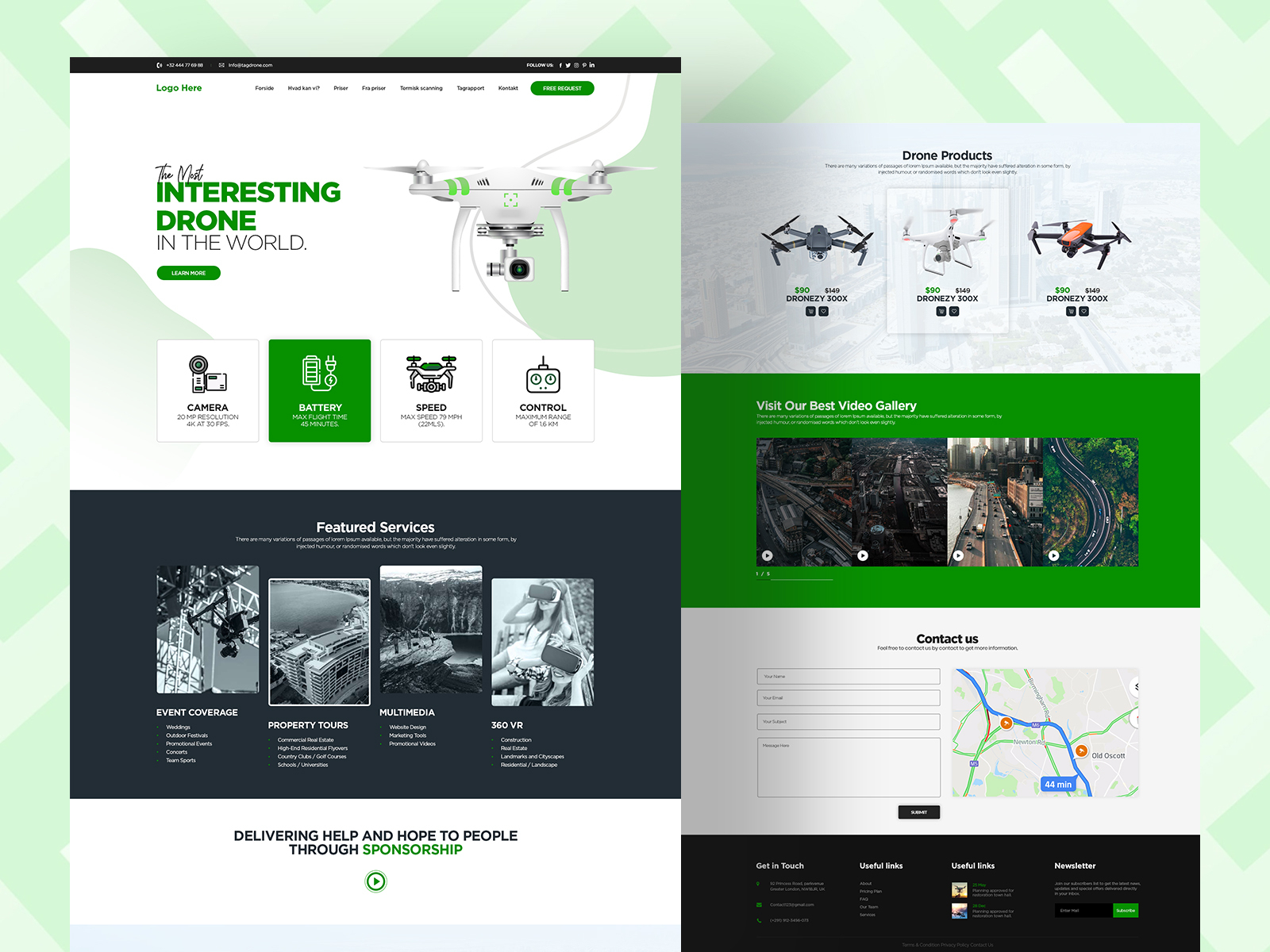The website displayed in the image features a detailed layout with a light green and dark green patterned background. On the left, there is a prominent section with several panels. The first panel is white and displays the text "Logo Here" at the top, followed by black print too small to read. Below this is a green banner with "Free Request," and at the bottom of the panel, "The Most Interesting Drone in the World" is highlighted with a "Learn More" button. Illustrating the product, an image of a drone is accompanied by labeled squares indicating its features: "Camera," "Battery," "Speed," and "Control."

Further down, a dark charcoal background with white text lists various services: "Feature Services," "Event Coverages," "Property Tours," "Multimedia," and "360 VR." Beneath this, on a white background with charcoal print, there is a message, "Delivering Help and Hope to People Through Sponsorship," where "Sponsorship" is notably highlighted in green text.

On the right side, three main panels are present. The top panel is gray and titled "Drone Products," showcasing three different drones. Following this, a panel with a bright green background invites visitors to "Visit Our Gallery – Best Video Gallery," featuring aerial views of various locations. The final section is the contact form, including fields for name, email, and a map, with additional text reading "Contact Us" and options for interaction. At the bottom of the page, set against a black background, the site provides links for "Get In Touch," "Useful Links," and a "Newsletter."

This website is an organized and user-friendly platform, effectively presenting information and engagement opportunities related to drones and their applications.